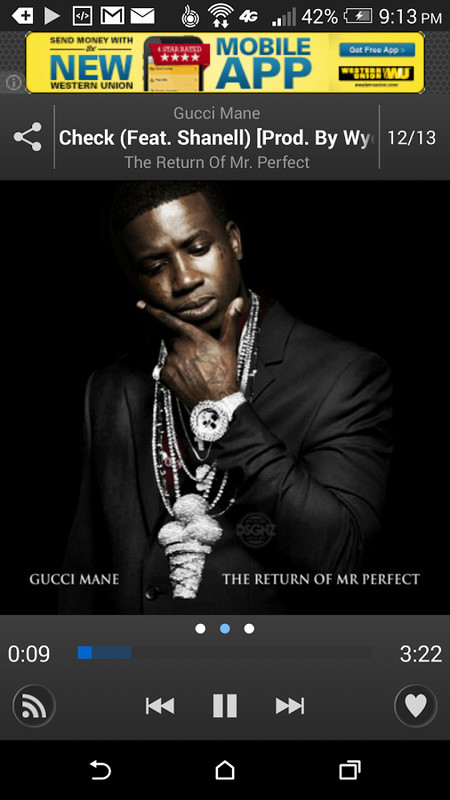Screenshot of a mobile app interface showcasing a song currently playing. At the top of the screen, a status bar displays various icons: the time (9:13 p.m.), battery status (charging at 42% with 2 out of 5 bars), 4G signal, Gmail and email icons. To the left, a horizontal yellow banner ad for the Western Union mobile app features bold blue uppercase text reading "SEND MONEY WITH THE NEW WESTERN UNION MOBILE APP," along with an image of a phone with a red banner stating "FOUR-STAR RATED."

Beneath the ad, the music player section shows a gray horizontal box with details of the song: "Gucci Mane - Check (featuring Chanel) [prod. by Y]" from the album "The Return of Mr. Perfect," identified as track 12 out of 13. Below this, an image of Gucci Mane is displayed; he is depicted wearing a dark gray suit with numerous silver necklaces, including one with a silver ice cream cone pendant. The text beneath the image reads "Gucci Mane - The Return of Mr. Perfect." The progress bar indicates the track is 9 seconds into its 3-minute and 22-second duration.